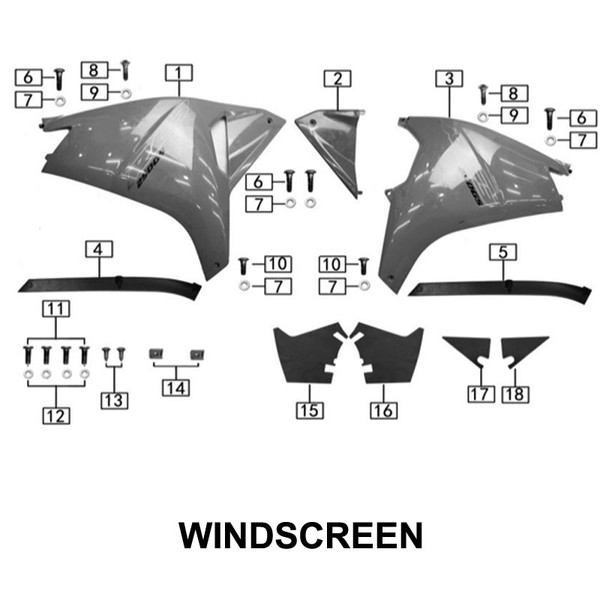The image is a detailed, grayscale diagram labeled "wind screen" in bold black text at the bottom. It appears to be an instruction manual or an assembly guide for a windscreen, possibly for an automobile or an aircraft. The diagram showcases a comprehensive, exploded view of all the components involved in the assembly, each meticulously numbered from 1 to 18. The parts include various screws, ringlets, metal pieces, corner pieces, and bars. Specifically, the numbers range as follows: several screws numbered 6, 8, 10, 11, and 13; ringlets numbered 7, 9, and 12; metal pieces numbered 1, 2, 3, 4, 14, and 16; a bar labeled 5; and corner pieces numbered 17 and 18. The image helps in identifying and understanding the placement and quantity of each part required for assembling the windscreen, illustrating a clear and organized view of the components.